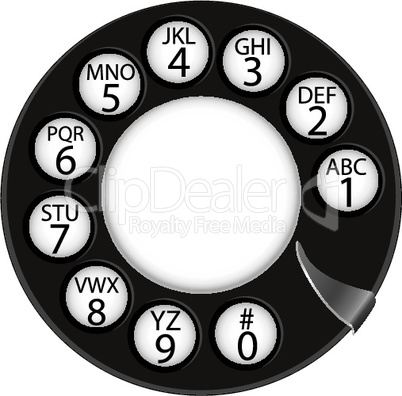This image features a detailed and accurately recreated close-up of an old-fashioned rotary phone dial, which appears to be computer-generated against a white background. The dial is primarily black with a white central circle, and distinct numbers and letters are inscribed around its circumference. Starting from the right side of the inner white circle and moving counterclockwise, the numbers progress as follows: 1 through 9 and 0. The number 1 is positioned on the right side, and each number is paired with letters: 1 (ABC), 2 (DEF), 3 (GHI), 4 (JKL), 5 (MNO), 6 (PQR), 7 (STU), 8 (VWX), 9 (YZ), and 0. Additionally, the number 0 includes a pound key (#). A small silver metal tab, serving as a finger stop, protrudes into the black circle on the bottom right. Inside the central white circle, the faint text "Clip Dealer, Royalty Free Media" is visible, extending slightly into the surrounding black area.